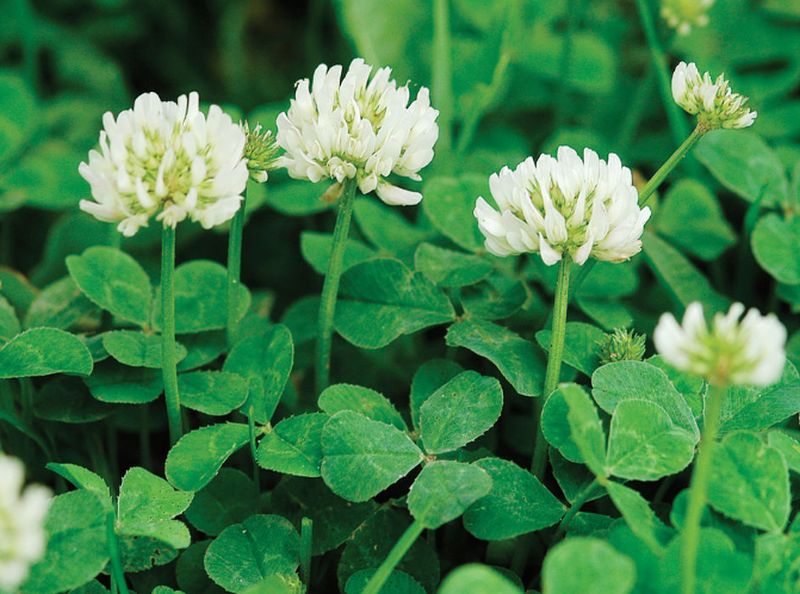This is a color, representational photograph taken outdoors during the daytime, depicting a close-up view of a green clover patch with multiple white flowering clovers. The image is in landscape orientation, approximately six inches wide and four to five inches tall. At the forefront, there are five distinct white clover blooms, each round in shape and attached to green stems with light tannish green bases. The central portion of the image prominently features three fully opened blossoms with multi-distinct white tips, surrounded by heart-shaped, green clover leaves. A partially visible white bloom is located in the lower left-hand corner, while another bloom is starting to blur out in the lower right-hand area. The overall background is a dark or black color, likely indicating the ground, and parts of the image, such as the top one-fourth and lower corners, exhibit blurred areas, focusing attention on the central clover flowers and leaves. The scene is a realistic portrayal of the natural beauty of flowering clover.